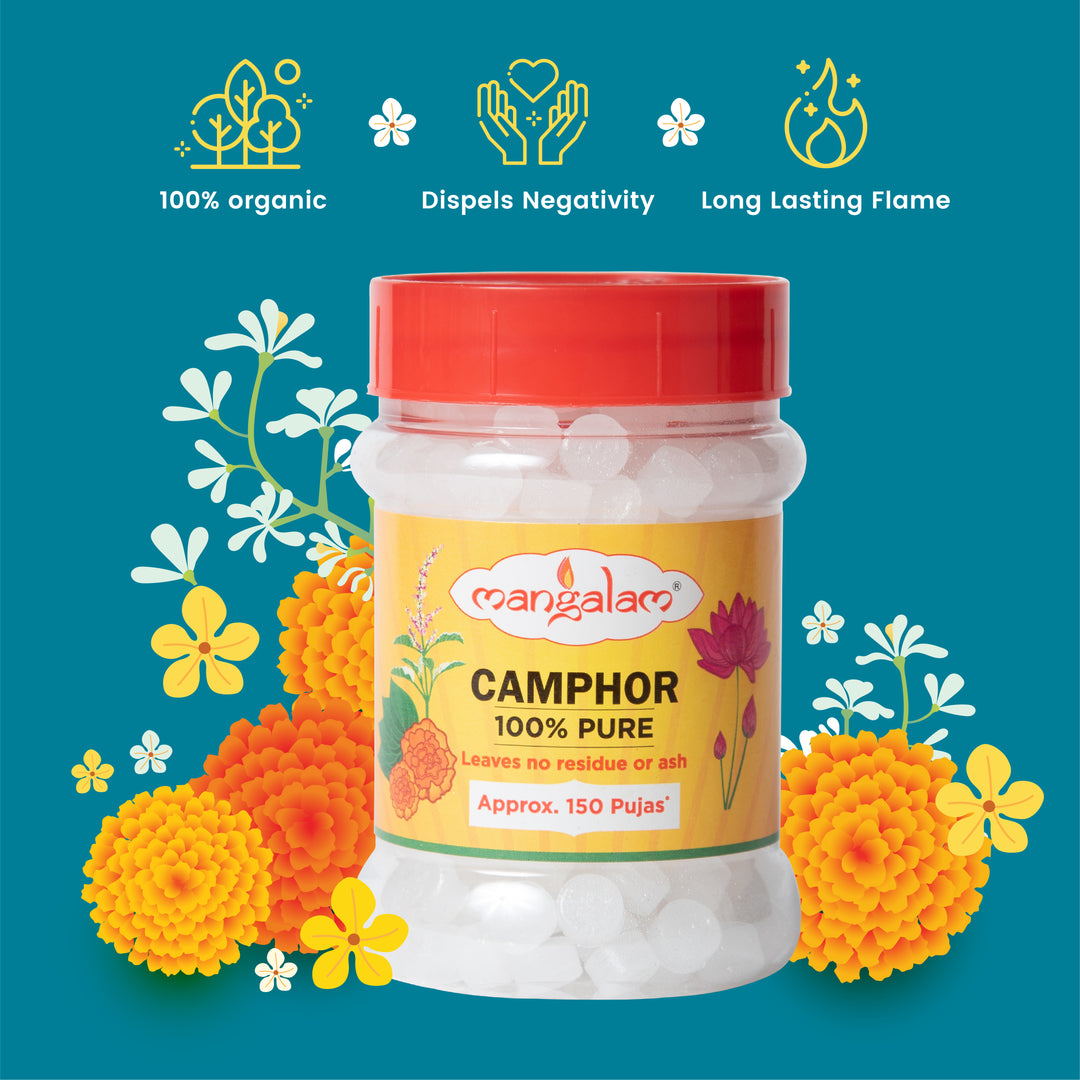The image showcases a product mock-up for a translucent plastic bottle with a red cap, prominently labeled "Mangalam" in black and orange lettering. This bottle contains pure camphor beads, described as 100% organic with properties of leaving no residue or ash, suitable for approximately 150 pujas. Above the bottle, three icons highlight its features: 100% organic, dispels negativity, and long-lasting flame. The bottle stands against a turquoise background adorned with clip art flowers in various colors, including yellow and orange marigolds, and white flowers with yellow centers, all featuring long green stems, enhancing the vibrant and spiritual essence of the product.